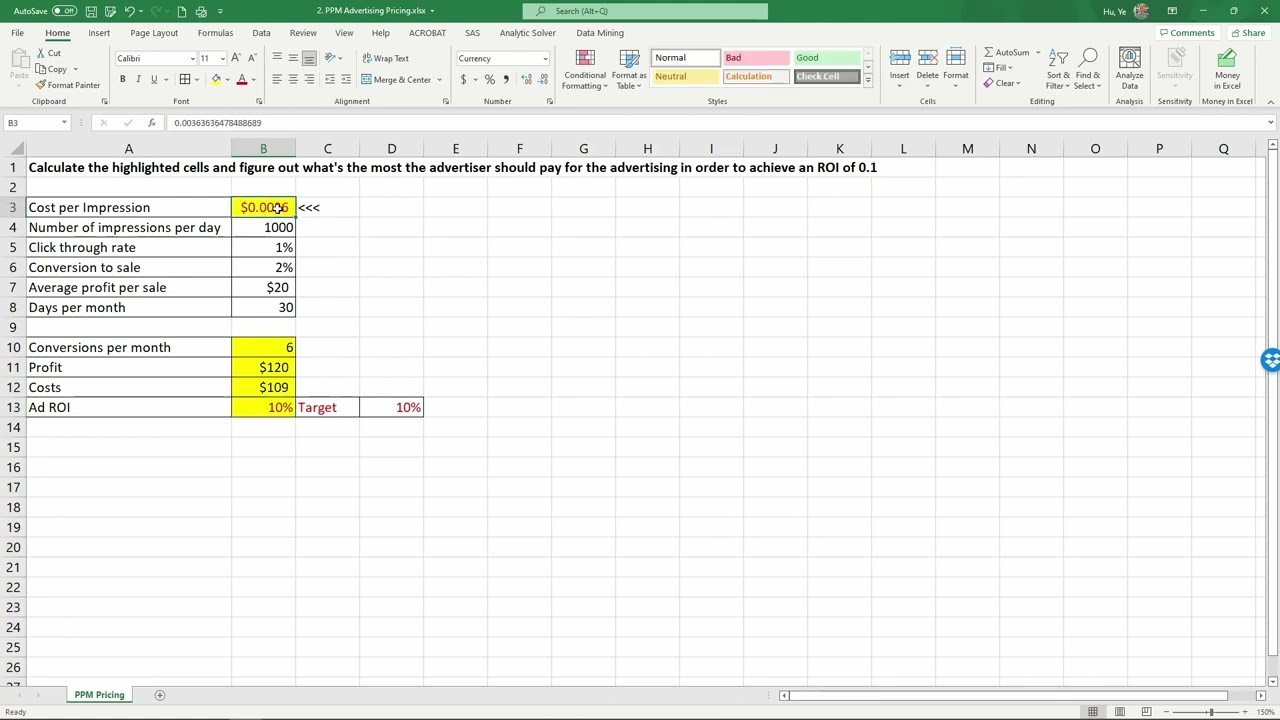The screenshot depicts an Excel spreadsheet containing a detailed setup for calculating advertising metrics. The interface exhibits the standard Excel features with a bright green taskbar at the top, providing options for various commands. The grid is organized alphabetically across columns (A to F) and numerically down the rows (1 through 27). Near the top, in bold black font, there's an instruction that reads: "Calculate the highlighted cells and figure out what's the most the advertiser should pay for the advertising in order to achieve an ROI of 0.1," where ROI stands for Return on Investment.

The spreadsheet includes rows titled "cost per impression," "number of impressions per day," "click-through rate," "conversion rate," "average profit per sale," "days per month," "conversions per month," "profit," "costs," and "ad ROI." Specific values are filled in to the right of these labels, with some cells highlighted in gold. Additionally, in red font, a target of "10%" is noted on the sheet. At the bottom left, the only tab visible is labeled "PPM pricing." The detailed structure and annotations suggest that this spreadsheet serves as a tool—possibly for instructional purposes—to determine the optimal advertising expenditure to achieve a specified return on investment.